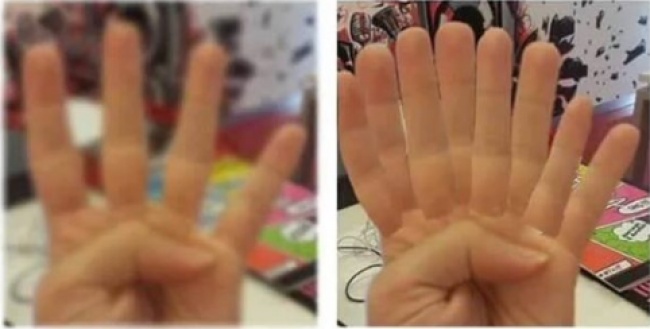The image features a side-by-side comparison of two photos depicting hands in different states of clarity. On the left-hand side, a grainy image shows a hand with four fingers extended and the thumb bent down towards the palm. The background is blurry, filled with indiscernible objects. In contrast, the right-hand side presents a much clearer image where the fingers appear to have multiplied, displaying eight fingers upright with the thumb also bent down towards the palm. The background here is more defined, revealing a paint-splattered wall with colors such as red, black, green, pink, orange, and white, as well as some cables and what seems to be a card or board game placed on a white surface. The juxtaposition of the images creates an almost illusory effect, emphasizing the bizarre multiplication of fingers in the clearer photo.